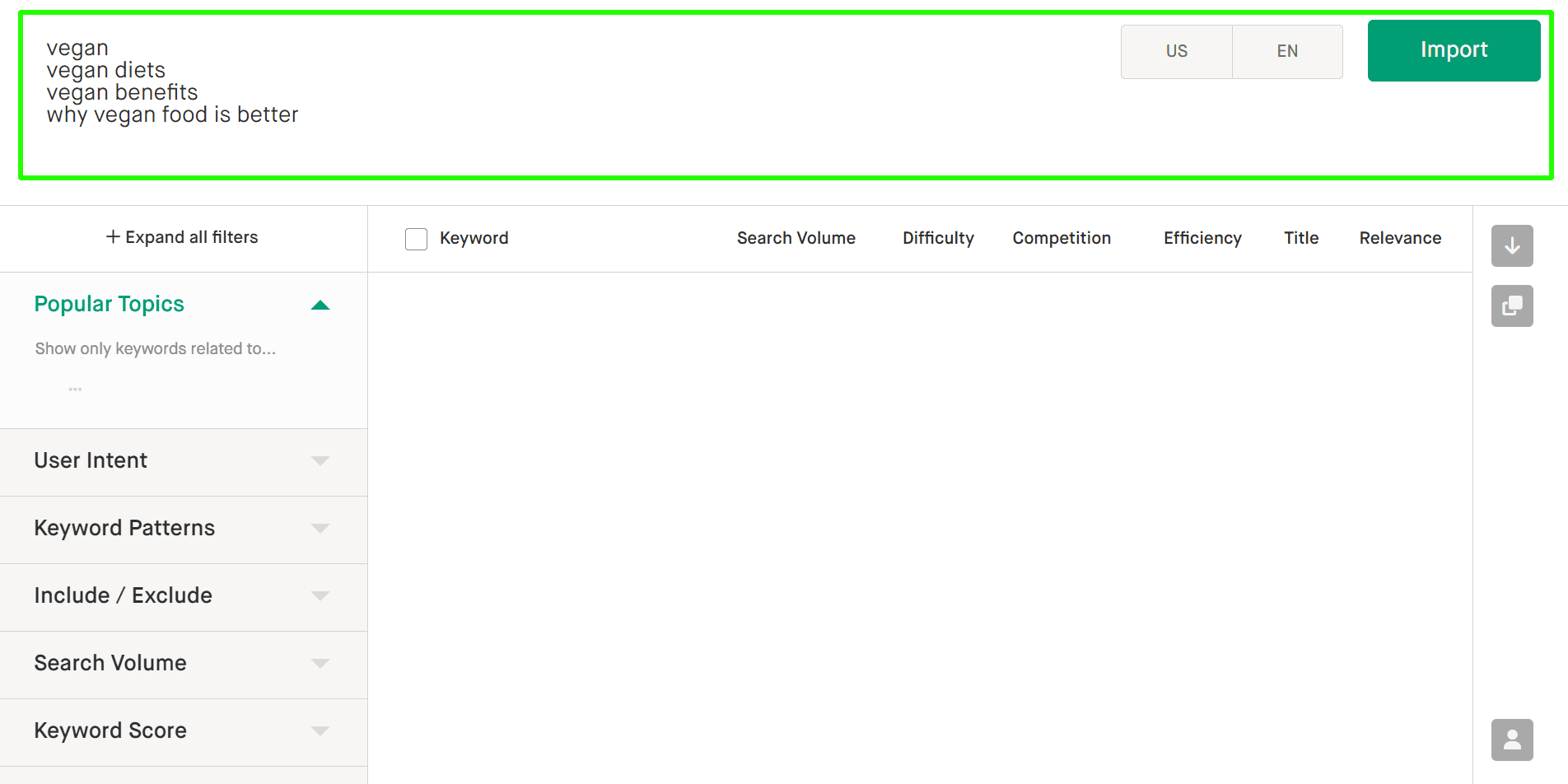The image features a user interface with a detailed layout. At the top of the image, there is a rectangular area bordered by a lime green line on all four sides. Within this rectangular area, the following text appears in successive lines: "Vegan," "Vegan Diets," "Vegan Benefits," and "Why Vegan Food is Better." 

To the right of this rectangular box, there are abbreviations "U.S." and "EN." Below these abbreviations, a dark green box labeled "Import" is present. Beneath the "Import" box, the text reads "Expand All Filters," followed by "Popular Topics" and "Show Only Keywords Related To." Further down, the text "User Intent" is displayed, detailing keyword patterns that include, exclude, search volume, and keyword score.

To the right of this section is a large empty white area with no content. Above this white space, there is a checkbox labeled "Keyword," which has been left unchecked. Adjacent to it, columns are labeled "Search Volume," "Difficulty," "Competition," "Efficiency," "Title," and "Relevance."